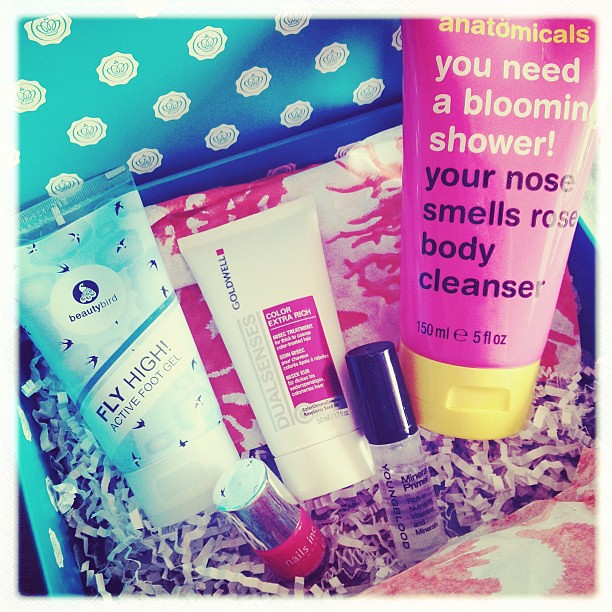This is a top-down view of a subscription box or gift kit filled with various self-care and beauty products. The box itself is blue, featuring shredded paper strips at the bottom which form a nest for the items inside. On the top right is the largest product, a pink tube with a yellow cap labeled "You need a blooming shower! Your nose smells rose body cleanser," containing 150 milliliters or 5 fluid ounces. To the left of this, there is a blue tube labeled "Fly Higher Active Foot Gel" from Beauty Bird, which features a circular logo at the top and the words "Fly High" on a white diagonal bar, capped with a white lid. Further left is a white tube, possibly from Goodwill, with a pink vertical rectangle and light gray rotated text, difficult to discern, also capped with a white lid. In front of these larger products, there are two smaller items: on the left, a metallic reflective bottle that appears to be nail polish in a dark pink shade with a silver lid, and on the right, a clear bottle with a black cap containing a clear liquid labeled "Mineral Primer" from Young Blood. The background of the box lid features a light blue interior with a white rose pattern, suggesting a thematic design element typically seen in curated beauty boxes.